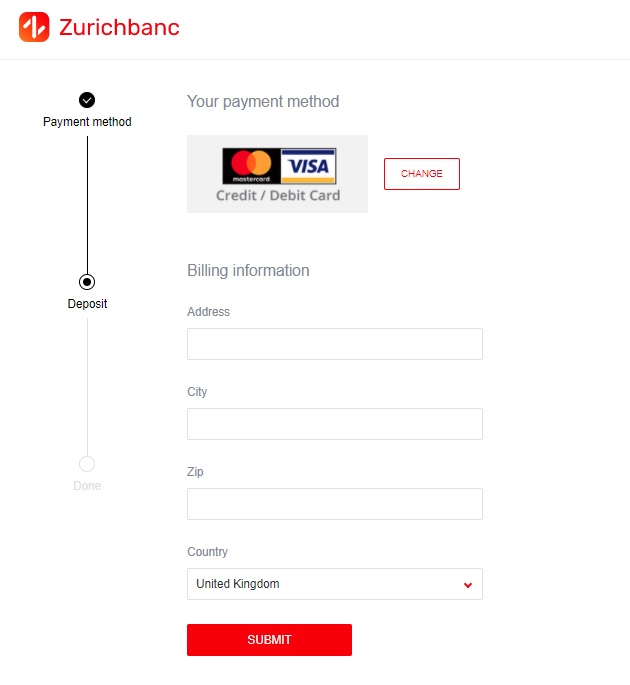**Image Description: Online Payment Page for Zurich Bank**

The image depicts an online payment interface for Zurich Bank. At the top, the Zurich Bank logo is prominently displayed, featuring a red square with a white 'Z' printed diagonally. Below the logo, the webpage title reads "Your Payment Method."

Under the title, there is a section to select the payment method, labeled "Credit or Debit." This section displays icons for MasterCard and Visa within a gray rectangular box. To the right of this box, the word "Change" is written in red and outlined in red, indicating the option to modify the selected payment method.

The following section is titled "Billing Information." Here, users are prompted to enter their billing details, including address, city, and zip code, each within separate white input boxes. The section also includes a dropdown menu for selecting the country, which is currently set to the United Kingdom. The dropdown arrow for changing the country is displayed in red.

To the left side of the image, there is a vertical step indicator for the payment process. The first step, "Payment Method," is shown as a black circle with a white check mark inside, indicating completion. A line extends downward to the second step, "Deposit," represented by a white circle outlined in black with a black dot in the middle, indicating the current step. Another line extends to the final step, shown as an outlined circle which is grayed out, signaling that it has not yet been completed.

At the bottom of the page, there is a prominent orange "Submit" button for finalizing the payment.

Overall, the structured and detailed interface provides a clear and organized method for completing an online payment.